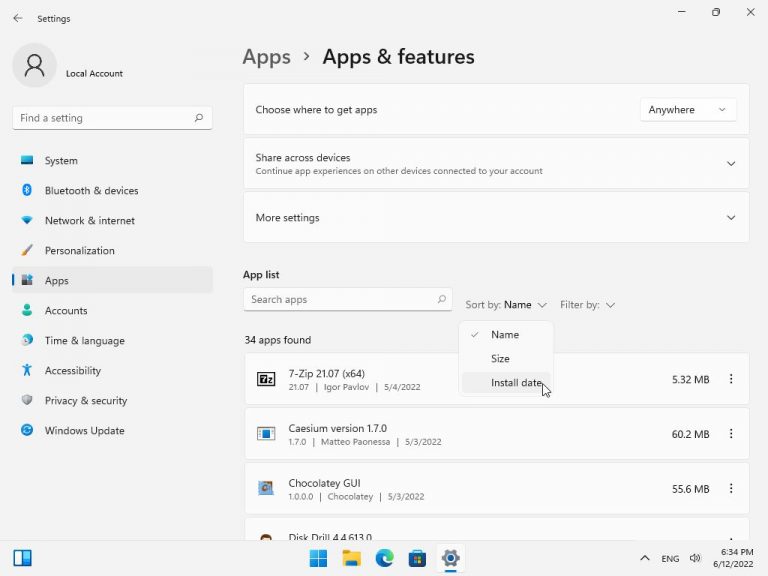This screenshot captures a desktop application's settings page against a grey background. At the top left corner, "Settings" is displayed in small black letters, with a left-pointing arrow next to it. Below this, there is a large circular icon displaying a stock image of a person's head, indicating the user profile area. To its right, the text "Local account" is displayed.

Beneath these elements lies a search box labeled "Find a setting," featuring a magnifying glass icon on the far right. Along the left side of the page, there is a vertical list of categories, including:

1. System
2. Bluetooth and Devices
3. Network and Internet
4. Personalization
5. Apps
6. Accounts
7. Time and Language
8. Accessibility
9. Privacy and Security
10. Windows Update

On the right side of the page, there's an exit button located at the bottom right corner.

In the central part of the screenshot, under the heading "Apps," "Apps & features" is prominently displayed in bold, dark print. Below this, there are three settings categories. The first category is labeled "Choose where to get apps," accompanied by a dropdown menu on the right side, which currently displays the option "Anywhere."

At the bottom of the page, a summary indicates that there are 34 apps found on the device. Additionally, information about the downloaded app's file size is provided.